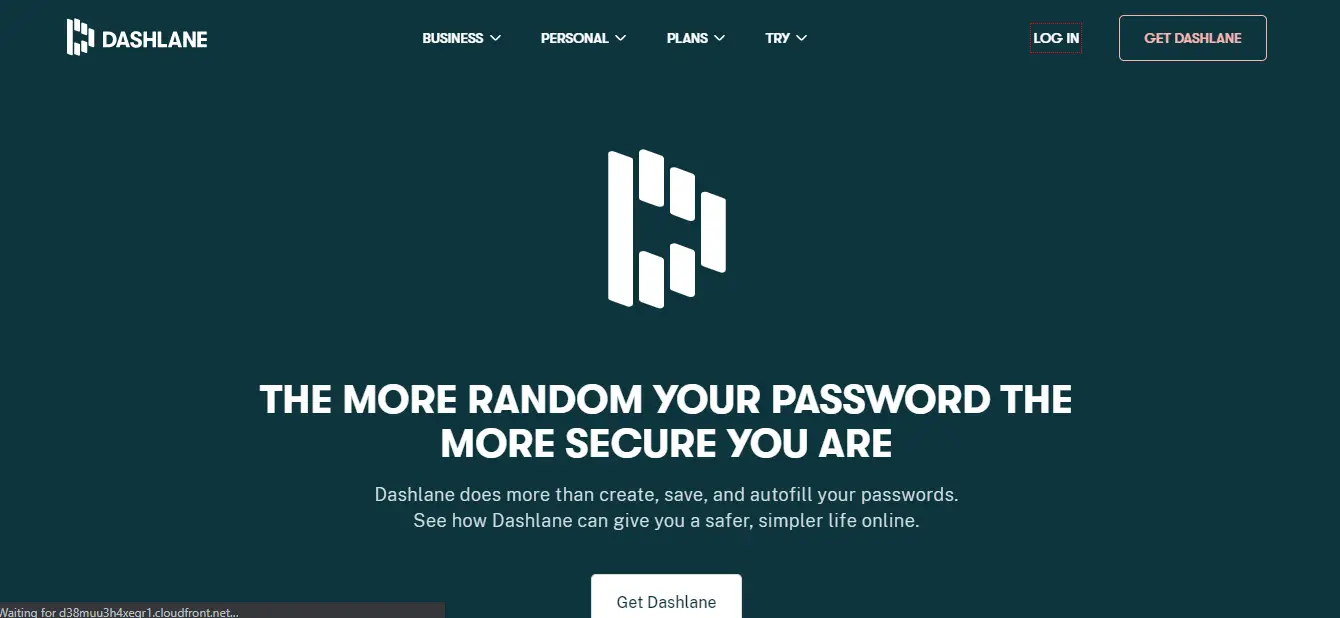The screenshot showcases the homepage of the Dashlane website, with a sleek and dark-themed design. 

- **Top Left Corner**: The Dashlane logo, an aggregate of individual rectangular shapes forming a 'D,' is prominently displayed.
  
- **Top Right Corner**: There are four navigation categories—Business, Personal, Plans, and Try—followed by a white “Login” option. Adjacent to these is a striking "Get Dashlane" button outlined in a pink rectangular border.

- **Central Section**: The central focus is the headline in large white font: “The more random your password, the more secure you are.” This is followed by a subtext in gray: “Dashlane does more than create, save, and autofill your passwords. See how Dashlane can give you a safer, simpler life online.”

- **Bottom Section**: Concluding the central visual area is another “Get Dashlane” button within a white rectangle featuring black text, inviting users to take action.

- **Overall Design**: The entire page is set against a sophisticated black background, offering a clean and modern user interface from top to bottom.